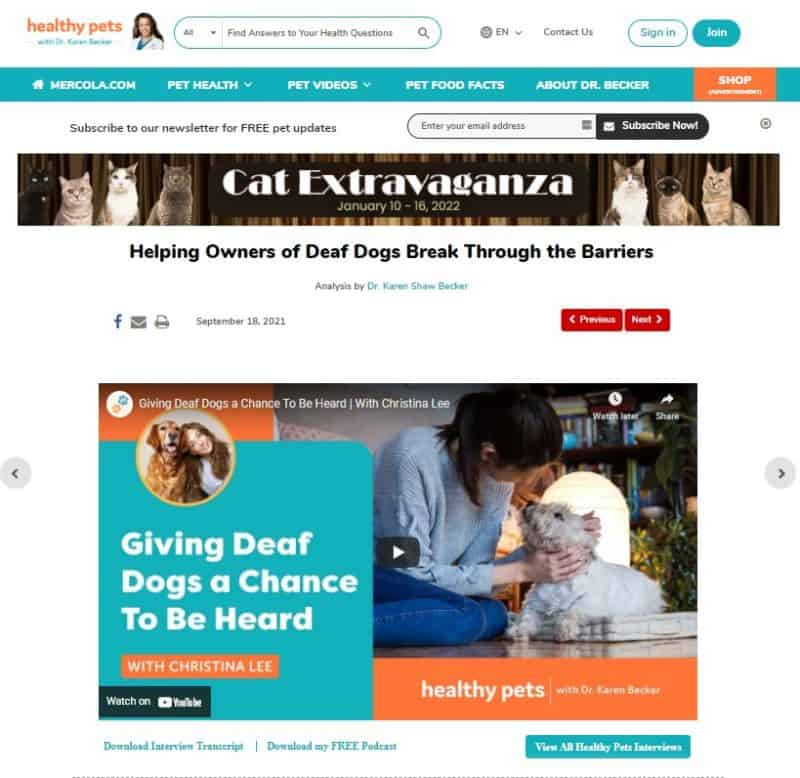This is a detailed and refined caption for the described image:

---

The web page displayed is from a site called "Healthy Pets," where the title "Healthy Pets" is prominently written in orange. The website features a vibrant and colorful design, primarily using shades of teal and orange. At the top of the page, there is a search bar labeled "Find answers to your health questions," a "Contact Us" link, a dropdown menu labeled "Ian," and options to "Sign In" or "Join," with the "Join" button highlighted in teal.

A teal-colored band at the top of the page displays the text "mercola.com pet health," and includes several dropdown menus: "Pet Videos," "Pet Food Facts," and "About Dr. Becker." An adjacent orange button allows users to shop. Below, there is a call to action to subscribe to a newsletter with the text "Subscribe to our FREE Pet Updates," inviting users to enter their email address and click "Subscribe Now," which is in black.

Beneath these elements, there is a section highlighting "Cat Extravaganza," featuring a bar with pictures of cats. Below, an area dedicated to assisting owners of deaf dogs is presented with the headline "Helping Owners of Deaf Dogs Break Through Barriers." An accompanying image shows a woman, Christina Lee, with her white deaf dog, both looking at each other. The caption mentions that Christina Lee is the host of this segment and provides an additional picture of her with another dog. Users are prompted to watch related content on YouTube. At the bottom of the page, there is a somewhat unclear link to view all pet insurance options, which needs improvement for better legibility.